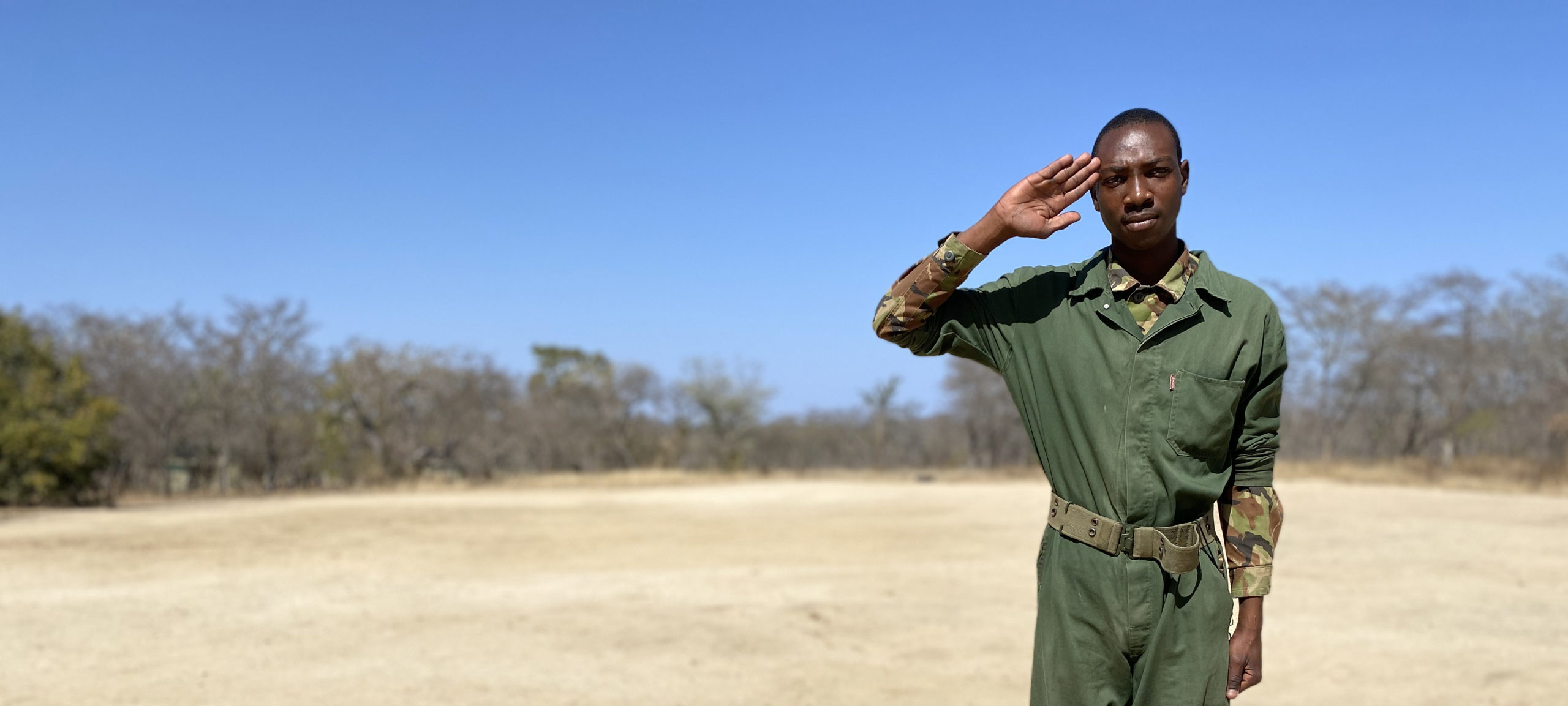In this vivid outdoor photograph, set on a bright day under an expansive blue sky, a black gentleman stands slightly left of center, saluting with his right hand, palm prominently visible. He dons a green military-style jumpsuit over camouflage fatigues in shades of black, brown, tan, and green, cinched at the waist by a vintage army belt reminiscent of those used from World War II to the Vietnam era. The background, mostly blurred, features an arid, sandy terrain devoid of plant life, and a row of trees stretching horizontally. While the leftmost tree is greener and clearer, those to the right are dry, mostly bare, and blend into the backdrop.